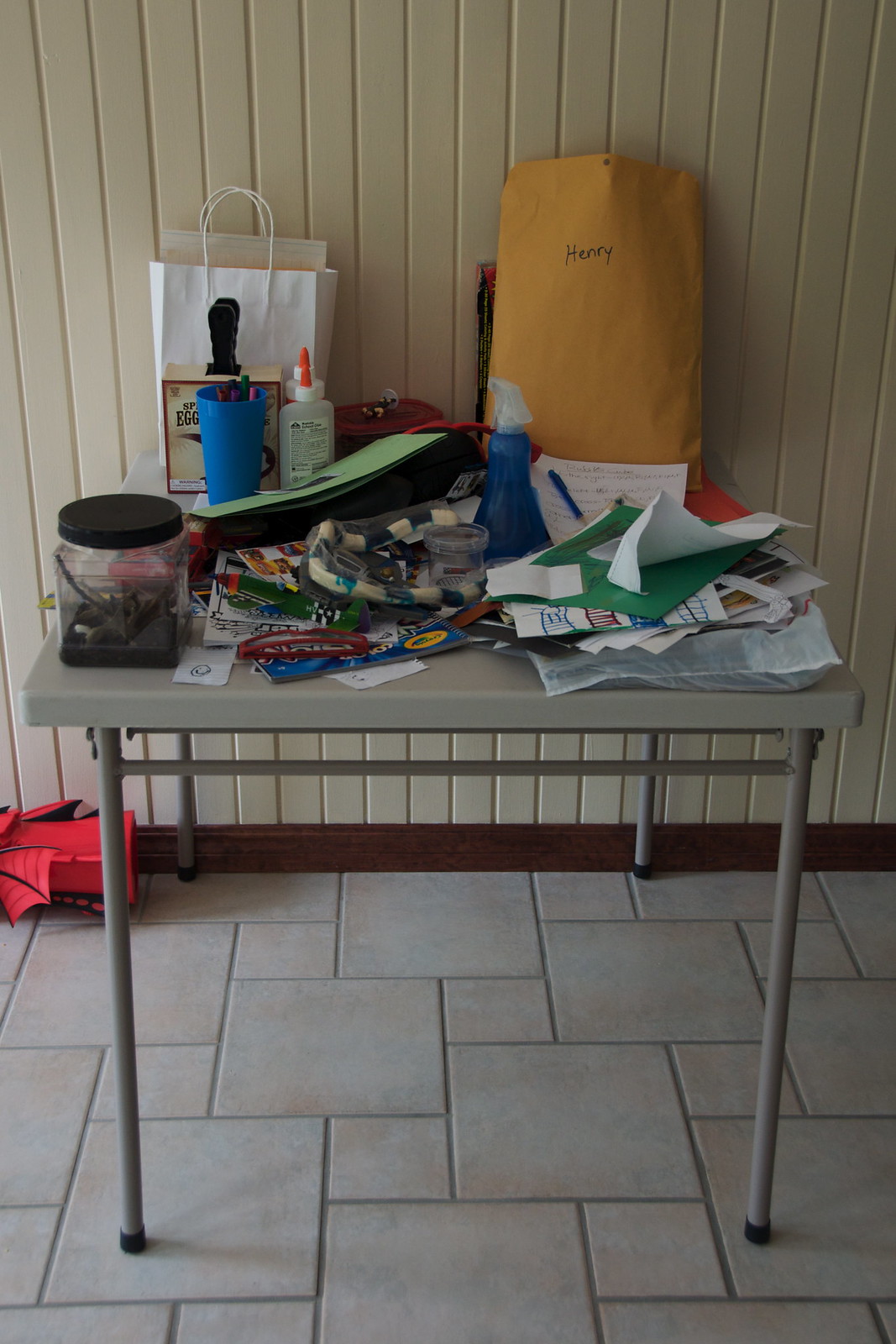The photograph showcases a gray table with black rubber legs, positioned on a gray tiled surface accented with gray grout lines. The table is cluttered with various items, each contributing to a scene rich in detail. Among the items present, there is a clear jar with a black lid and a bottle of glue featuring a white and orange lid. A blue cup containing several markers or pens adds a splash of color. A white paper bag with white handles is also placed on the table, alongside a green envelope and a red envelope, both providing a contrast of colors. Additionally, a blue spray bottle and a blue pen are noticeable amidst the assortment of white papers scattered across the table’s surface. A manila envelope with black writing intersperses the display further. Directly beneath the table, a red object with black accents is partially visible. The tile floor below casts the table's shadow, emphasizing the light source direction. Behind the table, several items are leaning against a tan wall with distinct tan lines, adding another layer of texture and depth to the image.